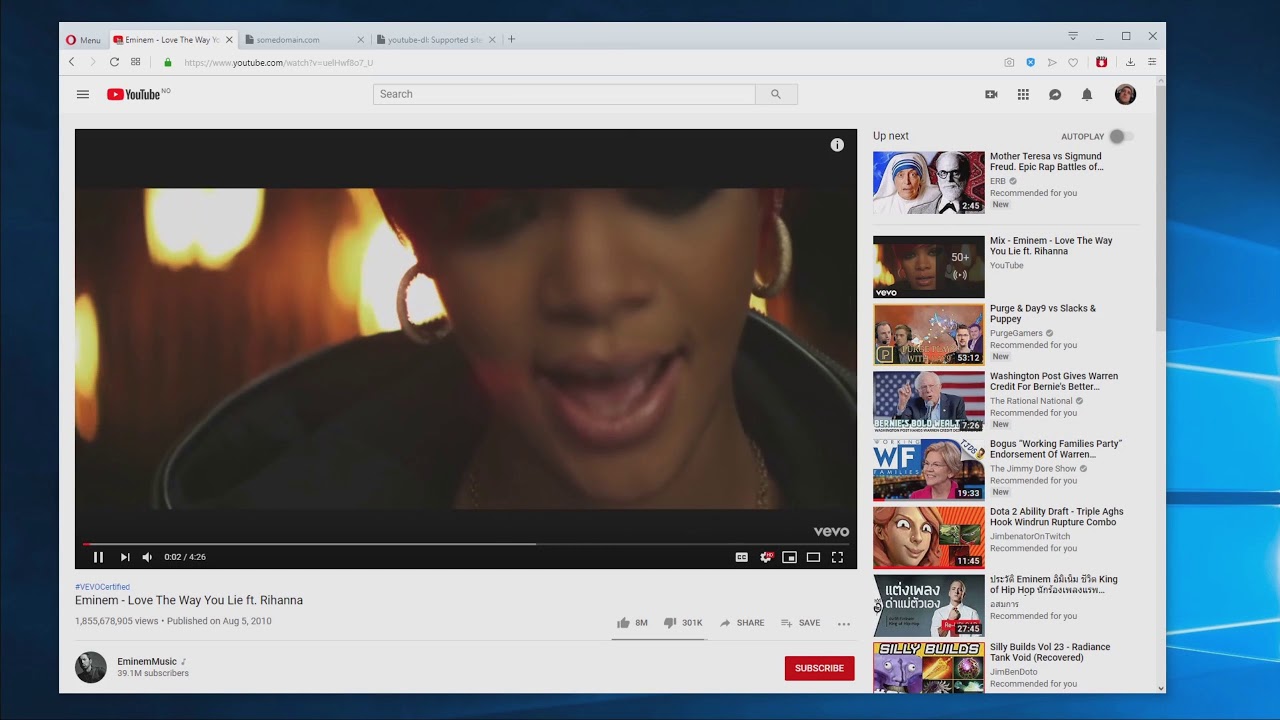Screenshot of a Traditional YouTube Desktop

This image captures a nostalgic view of an old YouTube interface on a desktop, set against a slightly off-gray background. The focal point of the screenshot is a music video featuring Rihanna, easily identifiable by the title and her appearance. Rihanna, of African-American descent, is seen singing with her signature black hair, adorned with gold hoop earrings, and dressed in a black sweatshirt.

In the top-left corner of the screen, there is a red circular icon with a white inner circle, labeled as "menu." Moving rightwards, the YouTube tab is displayed in its retro design with a red square housing a white right-pointing triangle and a small 'X' to close the tab. The partially visible title of the video tab refers to “Eminem, love the way,” which is cut off.

Adjacent to the YouTube tab, navigation arrows indicate browsing directions: a black arrow pointing left, enabling the user to go back, and a grayed-out right arrow, implying no forwards navigation is possible. The toolbar also includes a refresh icon, a grouped-square icon, and a green lock symbol, ensuring a secure connection.

The URL bar exhibits the address "http://www.youtube.com" followed by a unique watch identifier, "UELHWF807__U", all in capital letters. Below the video display, there is a certification text "Vivo certified" in blue, accompanied by a blue pound symbol. The video's title, "Eminem – Love The Way You Lie ft. Rihanna," is prominently displayed in bold black text, along with a view count of "1,855,678,905," a publish date of August 5th, 2010, total likes of 8,000,000, and 301,000 dislikes.

Interactive features such as the "Share" and "Save" buttons appear beneath the video. The player is set to HD, indicated by a small red square with "HD" in white lettering positioned at the lower left bezel of the video window. Below that, the channel name "EminemMusic" in black, garnished with a gray music note icon, reflects its 39.1 million subscribers. There is a red "Subscribe" button with white text inviting users to follow the channel.

To the right of the video player is a column filled with suggested videos. Another tab next to the active one displays a partially visible document icon labeled "somedomain.com" and "YouTube-DB support site," each with close button 'X'.

In the far-right corner of the browser window, several control icons include three ellipses for additional settings, a down-arrow for options, a minimize icon, a square to expand the window, and another 'X' to close the window. The overall desktop background is blue with a cyan blue Windows motif.